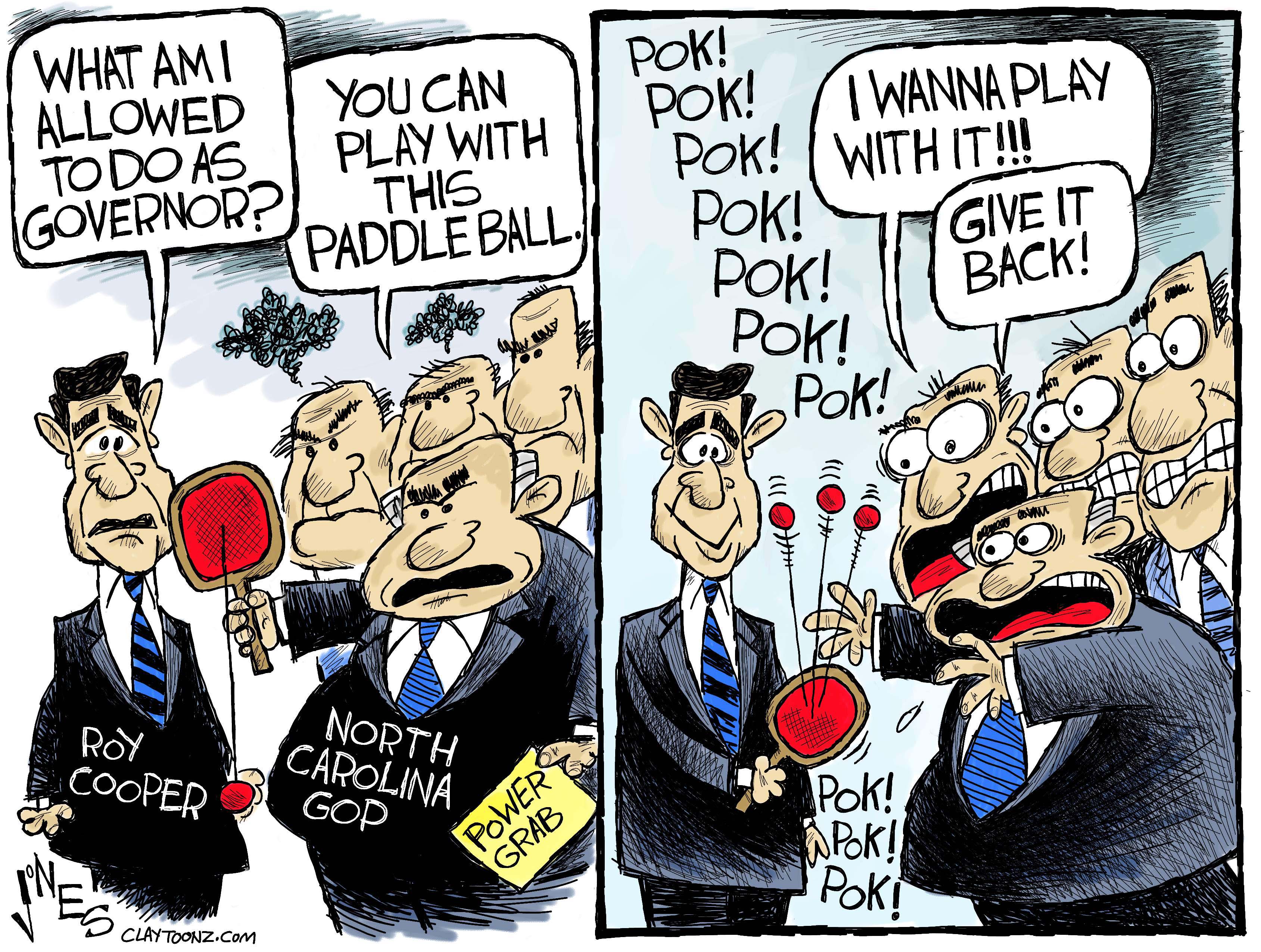In this two-panel political cartoon from claytoons.com, the left panel depicts North Carolina Governor Roy Cooper, dressed in a suit and a black and blue tie, being approached by four overweight, balding men in similar suits labeled "North Carolina GOP." The GOP members hold an envelope marked "Power Grab" and a paddle ball with a string. Governor Cooper, with a speech bubble that reads, "What am I allowed to do as governor?" is handed the paddle ball by the GOP, who sarcastically respond, "You can play with this paddle ball." 

In the right panel, Governor Cooper is depicted happily bouncing the paddle ball, with a series of "puck, puck, puck" sound effects emanating from the bouncing ball. The formerly composed GOP members now have frantic expressions, wide eyes, and outstretched arms as they desperately say, "I want to play with it! Give it back," trying to reclaim the paddle ball from him. The cartoon is characterized by a typical political cartoon style, with exaggerated and illustrative elements.